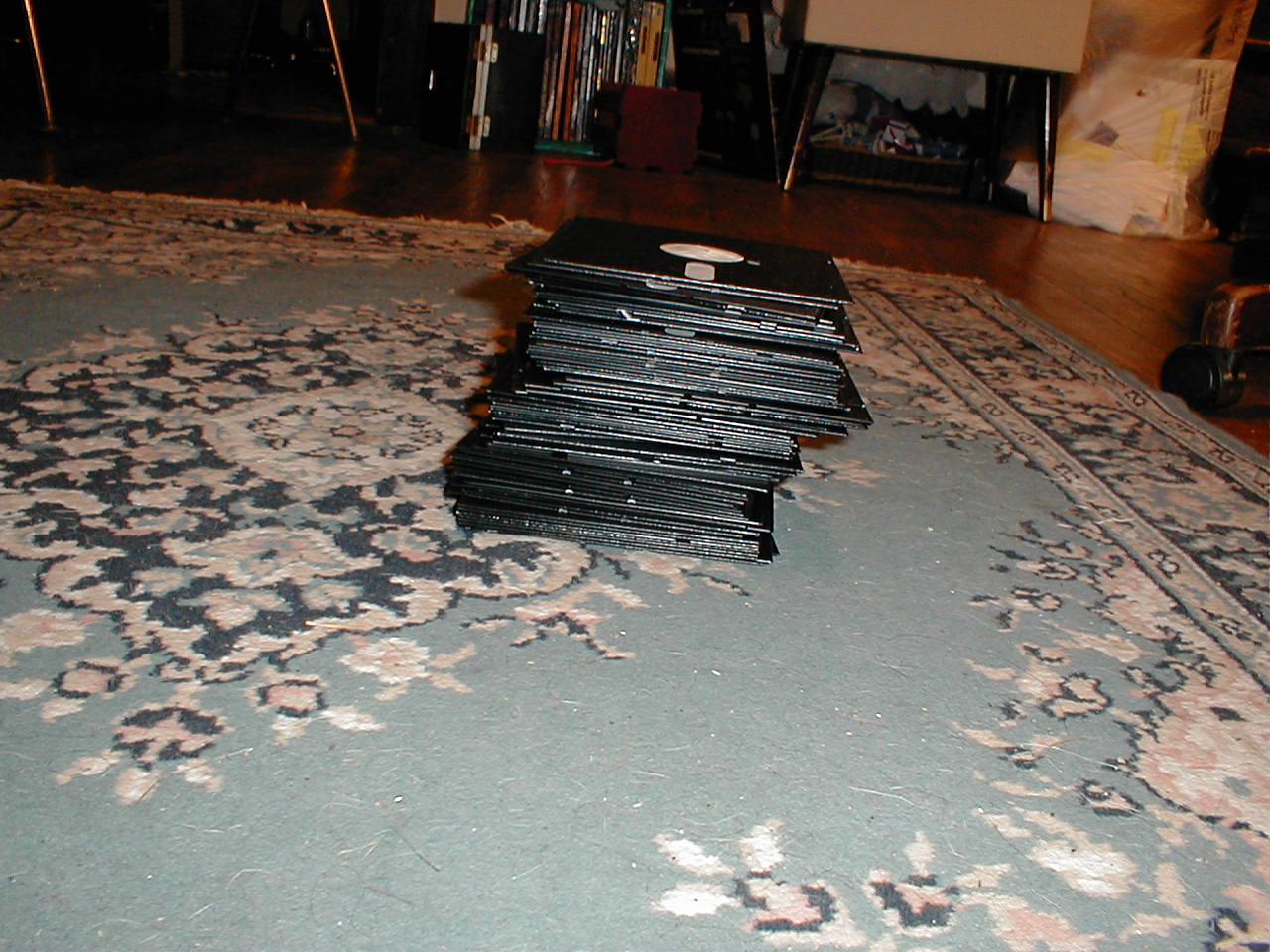A colored indoor photograph primarily focuses on a very worn and dirty oriental-style carpet that is tan and green, though it also has some blue sections with darker blue flower patterns. In the center of the carpet, there is a slightly tilted stack of approximately 25 to 50 black cardboard sleeves containing vinyl records. The topmost record's tan label is visible through the center hole of its sleeve. Surrounding the carpet, we see a dark wooden floor. Up against the left wall is a bookcase, though it's unclear whether it holds books or more records. To the right of the image, the legs of a couple of chairs are visible, and in the far corner, there is a clear plastic bag filled with what appears to be trash. The carpet is notably dirty, with visible pet hair scattered across it. The indoor photograph is well-lit with a flash and is in focus, capturing the lived-in and cluttered atmosphere of the living room.